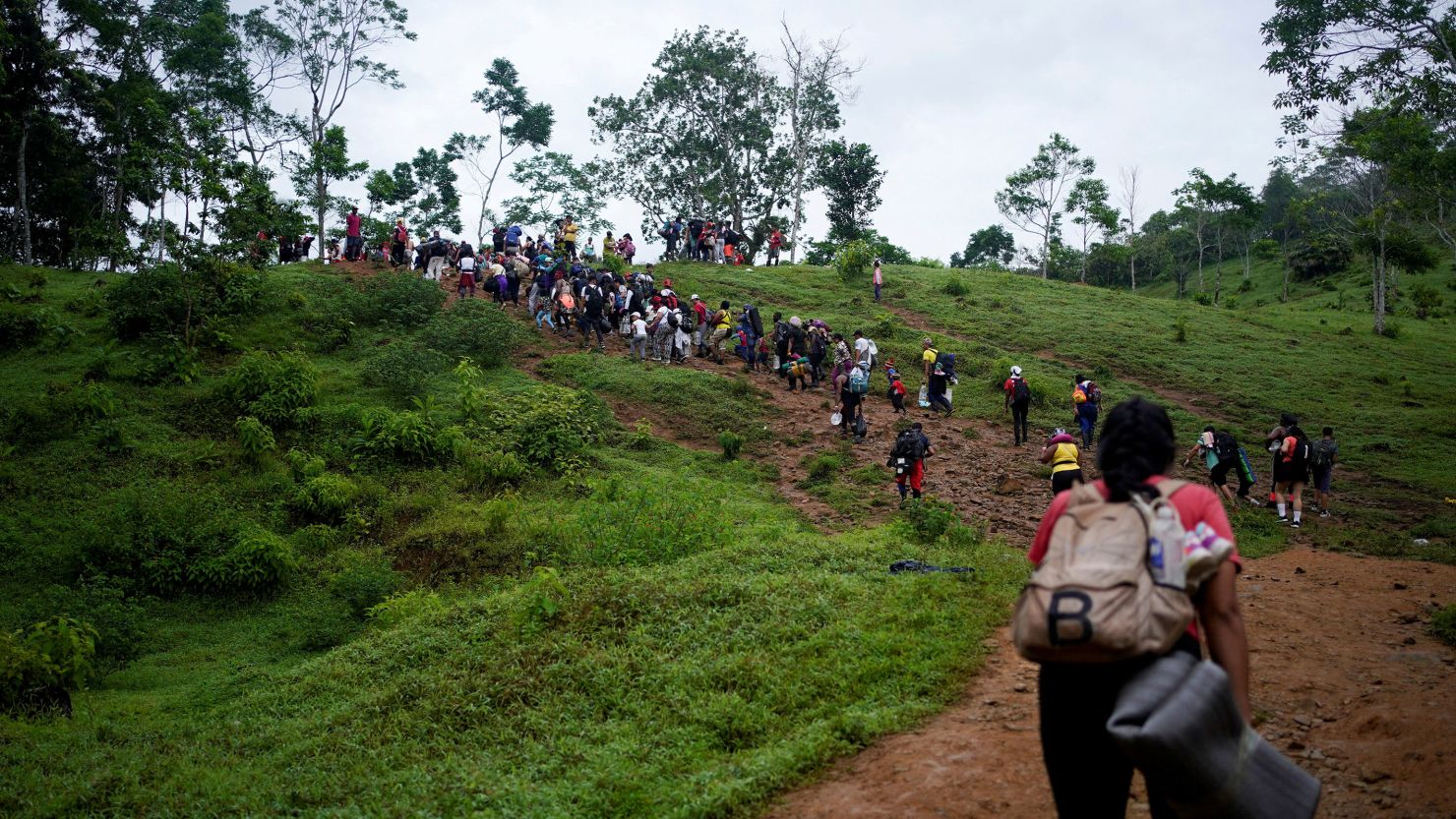In this image of the countryside, a large group of approximately 100 people is seen walking up a gently sloping hillside, possibly migrating to a new place. The slope, about a 15-degree angle, is covered with a dirt pathway flanked by green grass and bushes on the left, and just green grass on the right. These hikers are dressed in various colors and equipped with backpacks and water bottles. The surrounding landscape is richly green, populated with tall, slender trees and extensive vegetation. The closest to the camera is a darker-skinned woman wearing a pink shirt, short black hair, and a brown backpack with a prominent black letter "B." She carries a mat of some kind. Above them, a cloudy sky looms, adding a serene backdrop to their journey.